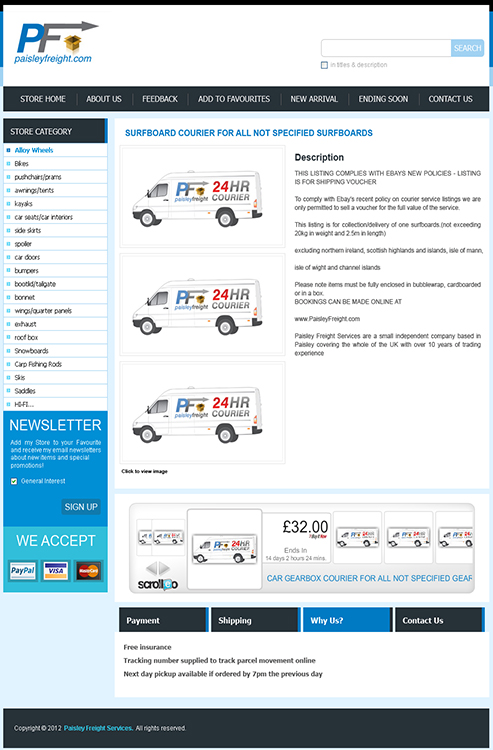This image is a vertically oriented rectangular graphic, featuring a detailed layout that seems to be part of a website or a digital storefront design.

In the upper left corner, a blue and gray "PF" logo is prominently displayed. The gray "F" has a unique horizontal top line that extends to the right, ending in an arrow pointing rightward. The top of the image is bordered by a black horizontal line that extends slightly down on both the left and right sides. This black line transitions into a vertical turquoise line, which then changes to a light blue line at the very bottom of the top section. Adjacent to the "PF" logo on a white background, there's a search box.

The main section of the page features several menus rendered in black with white, all-caps font. The menu items include: Store, Home, About Us, Feedback, Add to Favorites, New Arrival, Ending Soon, and Contact Us. Below the Store and Home tabs, there's another horizontal black box labeled "Store Category" in white, all-caps font. This section lists various items in black text, each preceded by a small turquoise dot. The top item in this list is highlighted in turquoise.

On the left, within a turquoise vertical rectangle, there is a section labeled "NEWSLETTER" in white, all-caps font, followed by some smaller text. Further down in this turquoise section, a message in white font indicates accepted payment methods, stating "We accept VIS, MasterCard, and PayPal."

The central part of the image is dominated by a bold turquoise title in all-caps: "SURFBOARD COURIER FOR ALL NON-SPECIFIED SURFBOARDS." Below this title, three white vans, each labeled "PF" and "24 HOUR COURIER," face the left edge of the image. 

Next to these vans, a section titled "Description" in black letters provides additional information, though the text is too small to be read. 

At the very bottom of the page, a price tag is displayed, possibly indicating British Pounds or Euros, marked at 32.